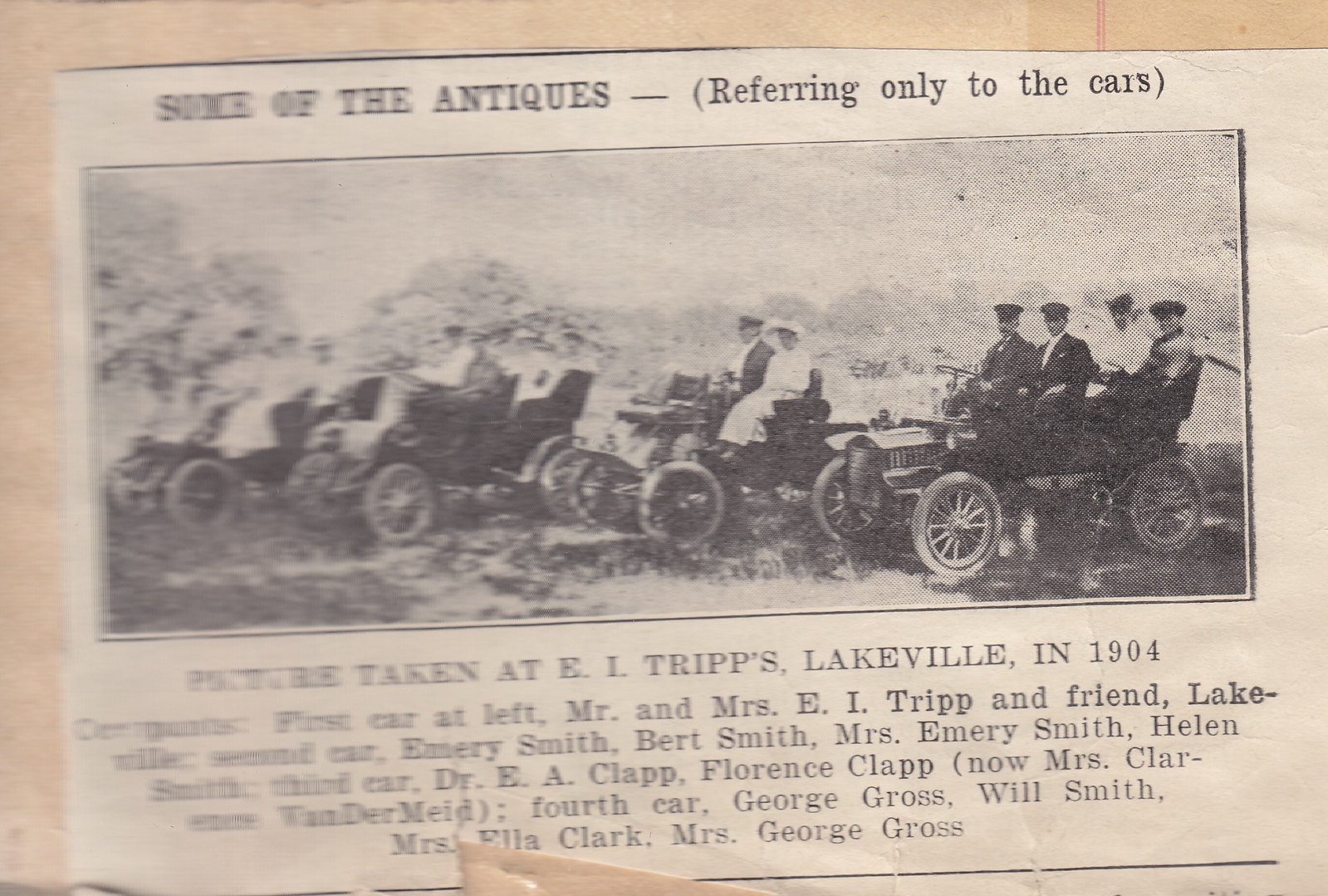The photograph is of an old newspaper clipping, affixed either to a brown paper bag or a lined, aged sheet, with its background showing distinct reddish lines. The clipping, in an off-white hue, appears to be glued or taped securely. At the top of the clipping, the caption reads, "Some of the antiques (referring only to the cars)," in black font. Below this, a rectangular, black-and-white photograph depicts four early 1900s automobiles, featuring wooden wagon wheels, parked on grass with various families and individuals inside. From left to right: 

1. In the first car, Mr. and Mrs. E.I. Trip and a friend from Lakeville, Indiana.
2. In the second car, Emory Smith, Bert Smith, Mrs. Emory Smith, and Helen Smith.
3. In the third car, Dr. E.A. Clapp and Florence Clapp, now Mrs. Clarson Vandermeade.
4. In the fourth car, George Cross, Will Smith, Miss Ella Clark, and Miss George Cross.

The left-hand side of the clipping is blurry, making it difficult to discern details, while the rest of the image is crisp and clear. The caption beneath specifies that the picture was taken at E.I. Trip's Lakeville in 1904. The entire montage provides a nostalgic glimpse into early automobile excursions, preserving a moment from over a century ago.